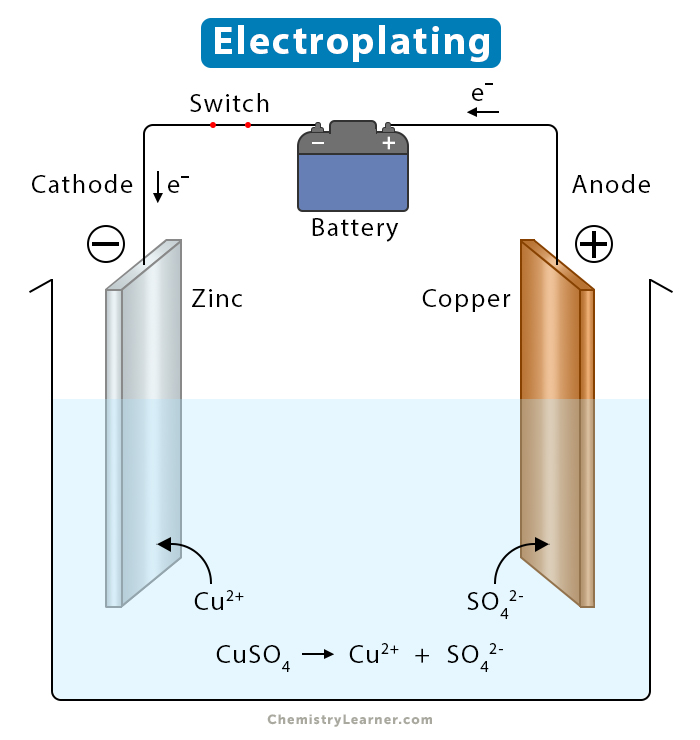This detailed illustration, possibly sourced from a scientific journal or educational site like chemistrylearner.com, demonstrates the electroplating process. At the top of the image, there is a blue rectangle with rounded edges containing the white text "Electroplating." Below this heading, a schematic shows a container filled with a light blue liquid, representing an electrolyte solution. Immersed in this solution are two electrodes: a gray one on the left labeled "Zinc" (Zn) and a brown one on the right labeled "Copper" (Cu). 

The zinc electrode, on the left, serves as the cathode, marked with a negative sign (-) and labeled "CATHODE." The copper electrode, on the right, serves as the anode, marked with a positive sign (+) and labeled "ANODE." A black and blue battery is illustrated at the top-center, with the positive terminal connected to the copper electrode and the negative terminal connected to the zinc electrode. Above the battery is a switch.

Scientific notations and arrows convey the direction of electron flow and chemical reactions involved in electroplating. Specifically, the diagram includes the chemical equation: \( \text{CuSO}_4 \rightarrow \text{Cu}^{2+} + \text{SO}_4^{2-} \). 

This diagram visually explains how zinc and copper are involved in the electroplating process, with zinc ions moving towards the copper electrode and plating it, illustrating the concepts of cathodes, anodes, and the overall mechanics of electrochemical reactions.